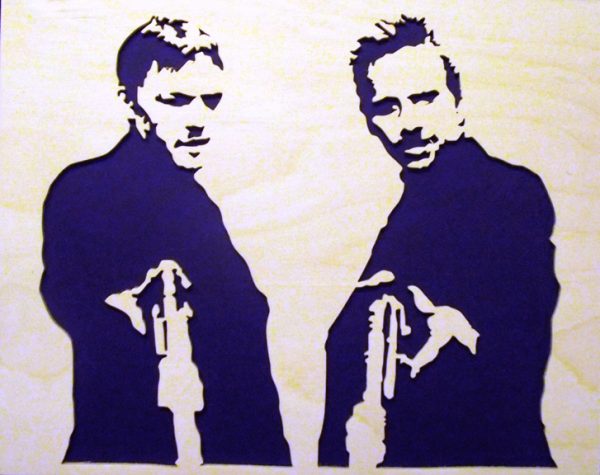This stylized illustration, reminiscent of a vintage film poster, portrays two men standing side by side against a faint yellow and white textured background. The image, primarily in black and white with a subtle bluish tint, appears to be a drawing or a photograph enhanced to resemble a drawing. Both men, likely white and wearing dark outfits, face the viewer with determined expressions while holding large guns, pointed downward but directed towards us. The man on the left holds his gun in his right hand and has neatly styled hair, whereas the man on the right, with slightly spiked hair, grips his gun in his left hand. The scene evokes a sense of tension and drama, reminiscent of a pivotal moment in a classic film, and draws a parallel to characters from a movie about two men seeking vengeance after a harrowing past involving Robert De Niro.